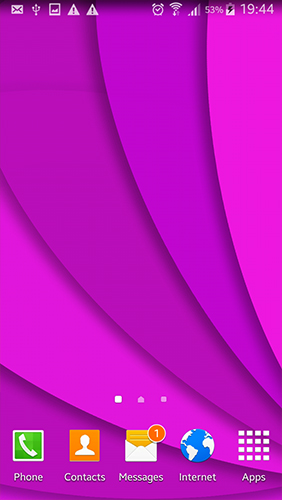This image captures a detailed screenshot of a cell phone background, showcasing various icons and interface elements against a visually appealing backdrop. The background is characterized by its swirling and semi-circular design with different shades of pink, transitioning from dark to light hues.

Starting at the top left, several icons are displayed in white: a male figure icon, a USB three-pronged port icon, a square image icon, followed by two yield signs with exclamation points. Moving to the top right, there's an alarm clock icon, a Wi-Fi icon with a down arrow indicating connectivity status, and cellular signal strength showing three out of four bars. The battery indicator displays a 53% charge with an accompanying icon depicting a half-white battery and a black charging symbol. The time is shown as "19:44."

The pink background features multiple concentric layers, with visible differentiation in shades suggesting depth. There appear to be five clear layers, with a hint of a sixth one. On the lower part of the screen, three white dots indicate navigation between home screens, with the left dot illuminated, suggesting this is the current screen.

At the bottom of the screen, a row of icons is visible:
- On the far left, a green phone icon labeled "Phone."
- Next, an orange icon for contacts labeled "Contacts."
- A white envelope with a yellow letter and an orange notification badge in the top right corner, indicating new messages, labeled "Messages."
- An old-style internet icon depicting a globe with white continents, labeled "Internet."
- Finally, an icon with multiple white squares, labeled "Apps."

This detailed arrangement and the aesthetic design of the phone's background and icons provide a comprehensive view of the user's interface layout and elements.